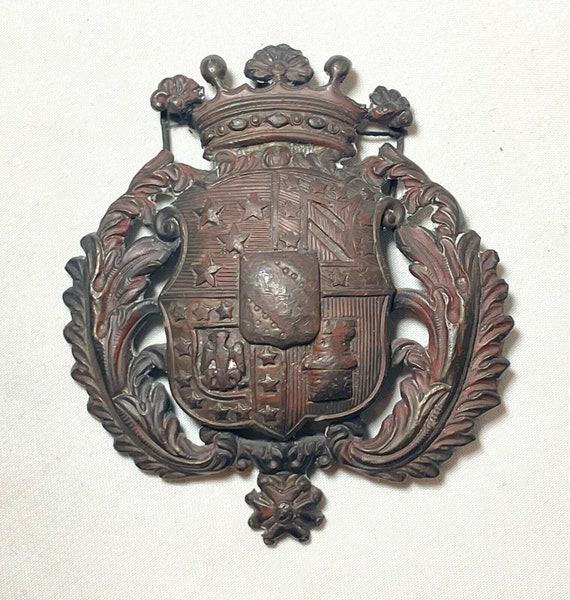This is a detailed color photograph of an antique metal crest, prominently displayed against a simple white cloth backdrop. The crest, seemingly an emblem or badge, is crafted from what appears to be steel, featuring a black base with a maroon tone and various shades of brown. At the center of the crest is a large shield, adorned with intricate etchings.

The crest is embellished with decorative elements: there are flowing ornaments resembling branches with leaves or fleur-de-lis on each side. At the very top, there’s a distinctive crown featuring two bulbous projections and three floral designs. 

Within the shield, the upper left corner showcases a cluster of stars, while the upper right corner displays a striped banner. The lower left corner features an eagle or bird with spread wings flanked by stars. Although slightly unclear, the lower right corner contains another object. Beneath the main emblem is a six-pointed star, adding to the intricate design. This three-dimensional crest, likely made of cast metal, gives the photograph a solid, tangible quality.